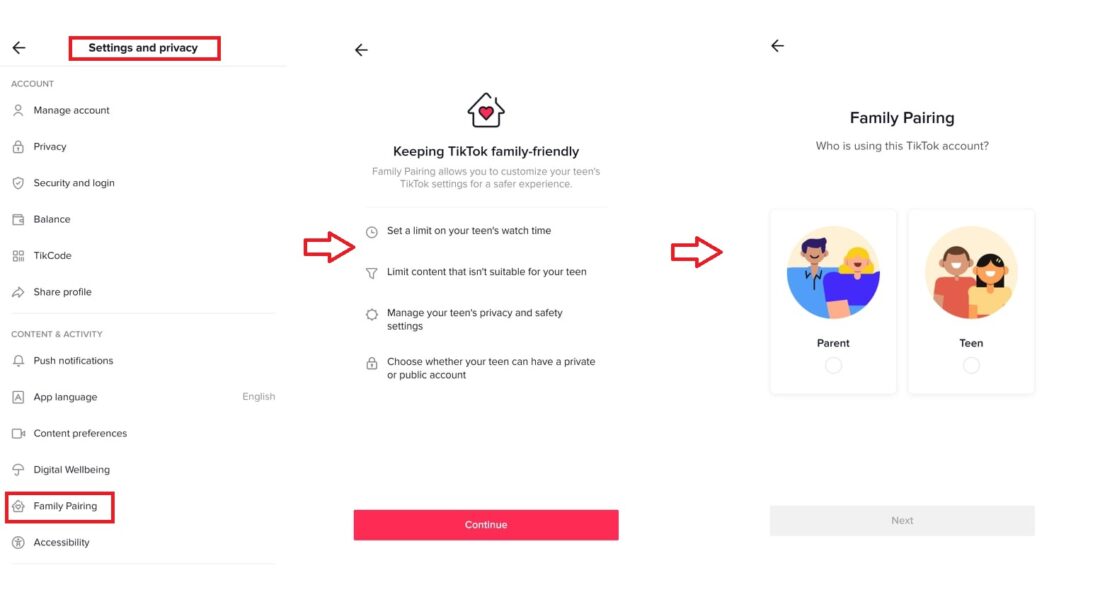**Detailed Caption:**

This composite image consists of three mobile screenshots placed side-by-side. 

- **Left Screenshot**: The interface displays the "Settings and Privacy" section, highlighted with a red box at the top. Below this, the screen is divided into two main categories: "Account" and "Content & Activity". Within "Content & Activity", "Family Pairing" is prominently shown, drawing attention with its placement. Additionally, a red arrow directs the viewer's attention towards the middle screenshot.

- **Middle Screenshot**: This screen is titled "Keeping TikTok Family-Friendly" and features an icon of a house with a heart inside it. The screen lists four crucial suggestions for parents: 
  1. Set a limit on your teen's watch time.
  2. Limit content that isn't suitable for your teen.
  3. Manage your teen's privacy and safety settings.
  4. Choose whether your teen can have a private or public account.
  At the bottom, there's a pink "Continue" button, and another red arrow points towards the rightmost screenshot.

- **Right Screenshot**: Titled "Family Pairing: Who is using this TikTok account?", this screen offers two avatar options. The first avatar, labeled "Parent", depicts a couple where the woman has blonde hair and wears a purple shirt, and the man has black hair and wears a blue shirt, all illustrated in a simple infographic style. Below it, the second avatar labeled "Teen" shows a sketch of two teenagers. A "Next" button is present at the bottom, but it is grayed out, indicating it's not currently selectable.

This detailed composition visually guides users through the family pairing setup process on TikTok, emphasizing parental control and safety settings.